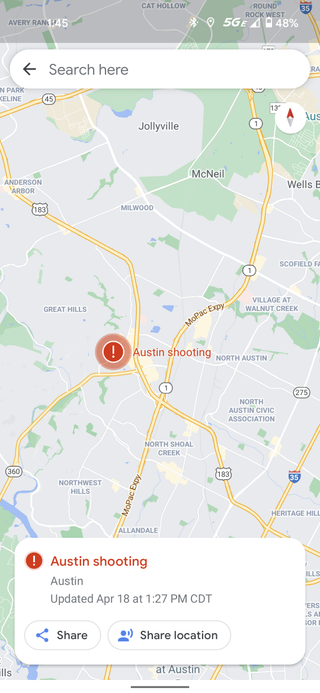Screenshot of a smartphone displaying a map of Austin, Texas with a notification about a shooting. The phone is connected to a 5G network and shows a battery level of 48%. The time is 1:45 PM. The map highlights the location of the incident with a red circle and an exclamation point, indicating a critical alert titled "Austin shooting." A pop-up on the screen provides additional details, stating the incident was last updated on April 18th at 1:27 PM Central Daylight Time. Below the notification, there are two buttons labeled "Share" and "Share Location." The map displays various city names in lighter colors, akin to a typical Google Maps interface.